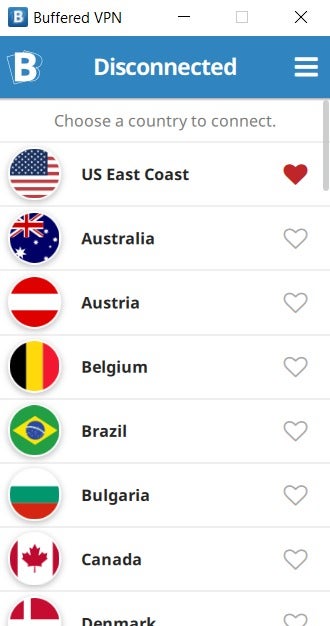The top left corner of the image contains a series of icons including a letter "B" positioned about four units away from a minus symbol within a square, an "X", and another "B", seemingly disjointed from surrounding elements. Next to these, a hamburger menu icon is visible. Beneath it, a selection prompt reads "Choose a country to connect," followed by a list of countries each accompanied by a flag and a heart icon indicating selection status.

- **United States (East Coast):** Represented by the American flag, with a solid (filled) heart icon.
- **Australia:** Shown with a flag featuring the Union Jack, and a hollow (unfilled) heart icon.
- **Austria:** Depicted with a flag consisting of red stripes on the top and bottom, and a white stripe in the middle, accompanied by a hollow heart icon.
- **Belgium:** Flag displayed with vertical black, yellow, and red stripes, alongside a hollow heart icon.
- **Brazil:** Featuring a green flag with a yellow diamond and blue circle in the middle, and a hollow heart icon.
- **Bulgaria:** Flag shown with horizontal white, green, and red stripes, and a hollow heart icon.
- **Canada:** The flag has red stripes on the left and right edges with a white center featuring a red maple leaf, paired with a solid (filled) heart icon.
- **Denmark:** The image includes a Danish flag, though specific details are overshadowed by a large bar at the top of the display.

The image as a whole appears to be a screenshot or interface of a VPN software, highlighted by the country selection feature and the visibility of internet connectivity options.